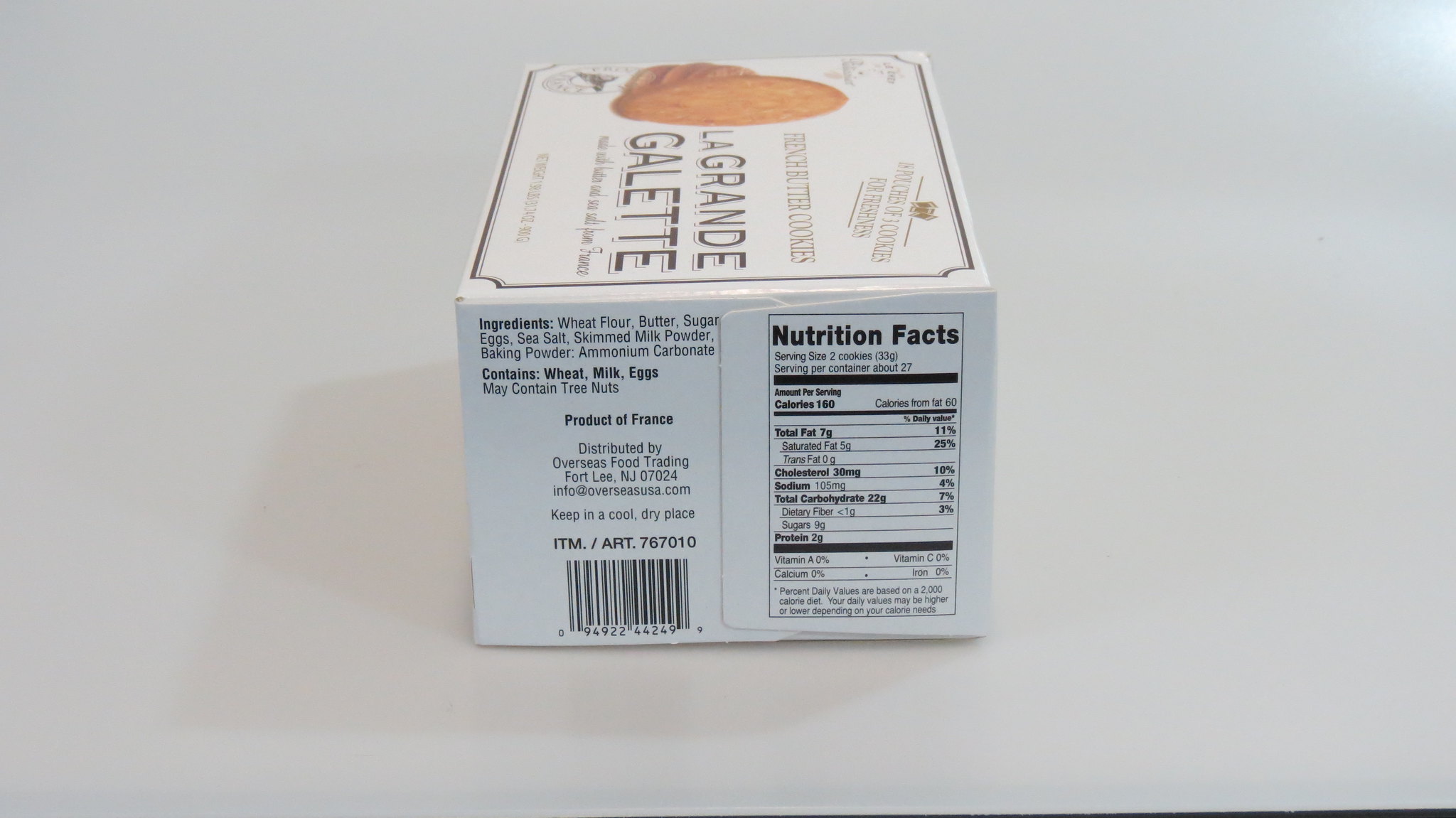The image showcases a box of LaGrande Galette butter cookies. The packaging prominently features the brand name "LaGrande" and the product name "Galette," which suggests these are a type of gourmet cookie. The ingredients listed include wheat flour, butter, sugar, eggs, sea salt, skim milk powder, baking powder, and ammonium carbonate. The product contains wheat, milk, and eggs, with a caution that it may contain tree nuts. In very fine print at the top, the label identifies these as butter cookies. Displayed on the upper section of the packaging is an image of an oval-shaped, smooth butter cookie, emphasizing its quality and appeal. Nutritional information indicates that each serving size of two cookies contains 160 calories. The product is distributed by Overseas Food Trading in Fort Lee, New Jersey 07024. A barcode is visible along with a white box containing the words “LaGrande Galette” and “gourmet sugar cookies.” The box itself is set against a light gray background, highlighting its elegant and sophisticated design.